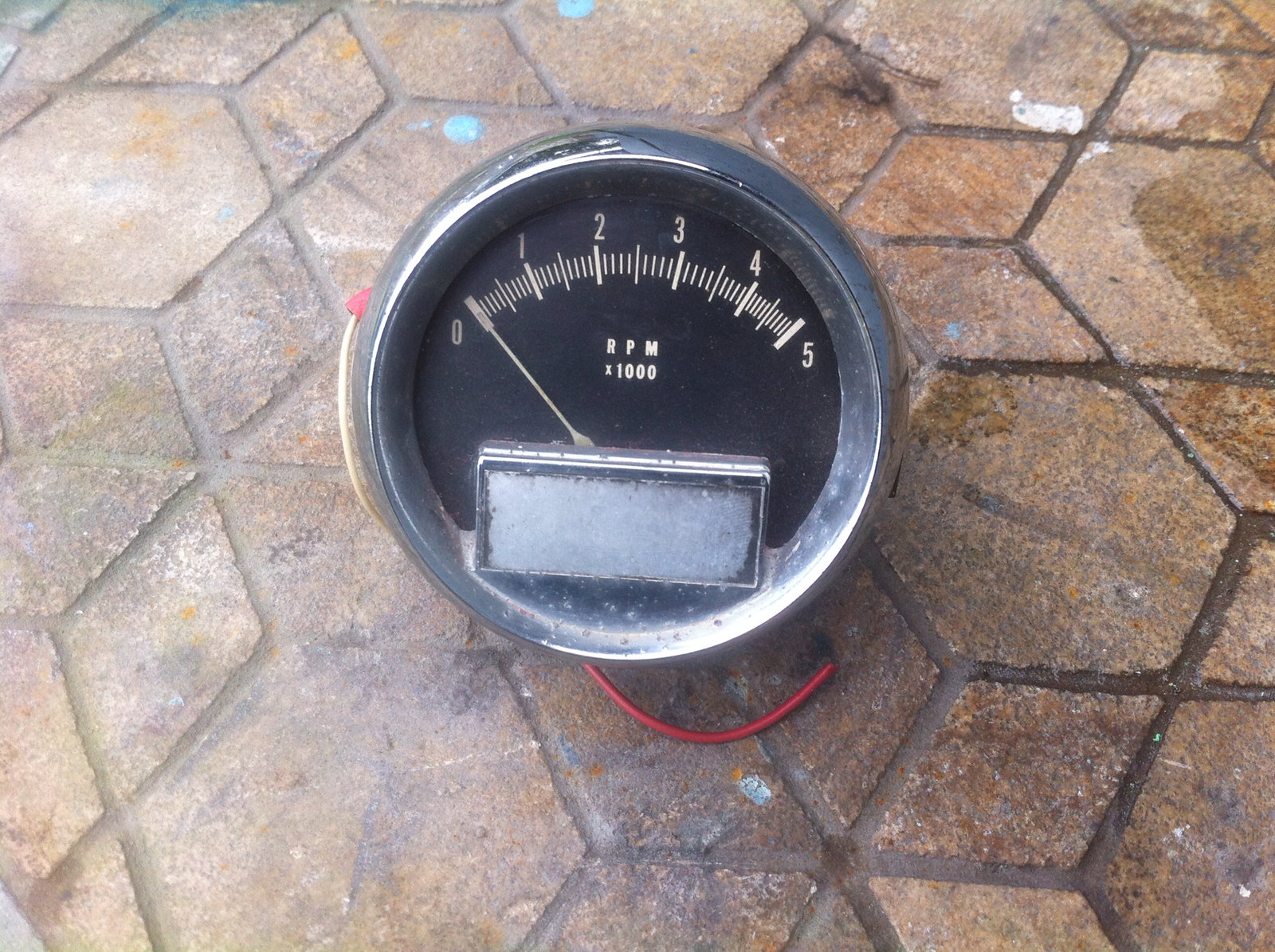A brown, concrete sidewalk composed of trapezoidal and diamond-shaped tiles stretches into the frame. At the center of the image lies a metal circular gauge, its face a stark black. The gauge displays numbers from zero to five, with "RPM x100" inscribed beneath, indicating rotations per minute multiplied by 100. A red cord extends from the gauge, suggesting its connection to another device, while a yellow cord is partially visible, snaking behind it. The gauge’s needle, colored white like the numerals, emerges from a metal rectangle at the bottom, poised to measure and indicate readings.